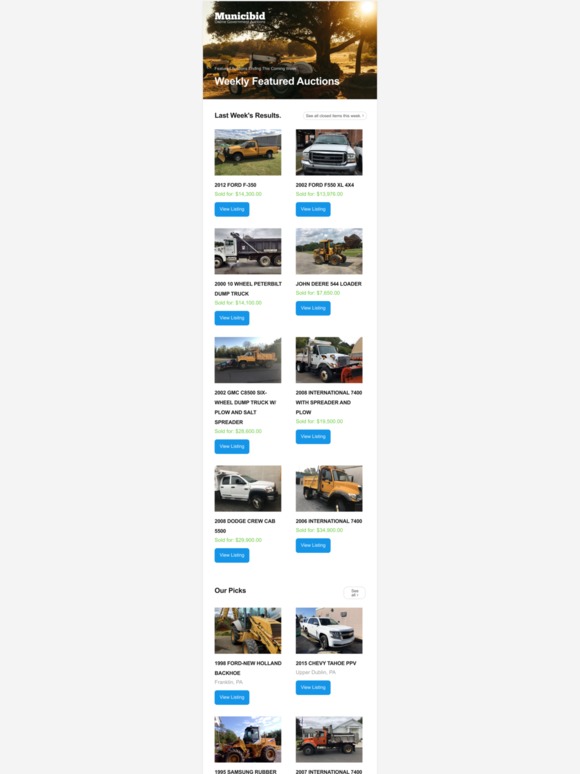The screenshot features a visually appealing, outdoor daytime scene captured at the top. The color photograph showcases a picturesque woodsy landscape with a large tree, behind which stands a structure that resembles a home or a barn, nestled amidst rolling hills lush with greenery. The sun peeks through the upper right corner, adding a warm glow to the serene image. Overlaid text in the upper left reads "weekly featured auctions" and "municibid."

Below the photo, the screenshot displays images of various auctions. The top left corner features an orange 2012 Ford F-350 truck. Adjacent to it in the top right is a white Ford F-350 XL vehicle. The row beneath displays a 10-wheel Peterbilt dump truck on the left and a John Deere 44 loader on the right. The final row features a 2002 GMC wheel dump truck, equipped with a plow and salt spreader, on the left.